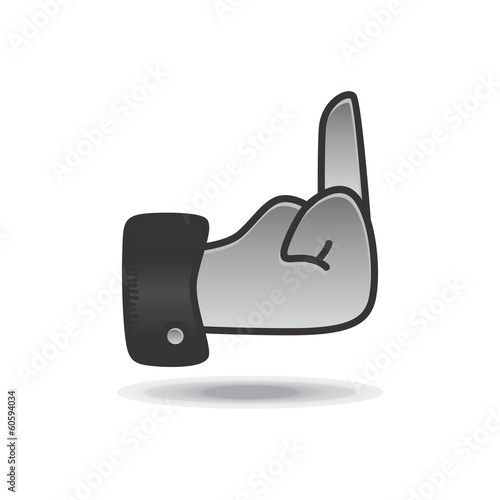In this black and white cartoon illustration, a hand is prominently displayed in the center, appearing to flip someone off with the middle finger raised. The hand, rendered in varying shades of gray, is outlined in heavy black lines. The sleeve from which the hand emerges is a dark gray with a distinct cuff and button, adding detail reminiscent of a jacket. Below the hand, a shadow transitions from dark gray at the center to lighter gray at the edges, creating a sense of depth. Diagonally across the background, the words "Adobe Stock" are faintly repeated, indicating a copyright watermark. Additionally, small print along the side of the illustration reads "Adobe Stock, line number 60594034."